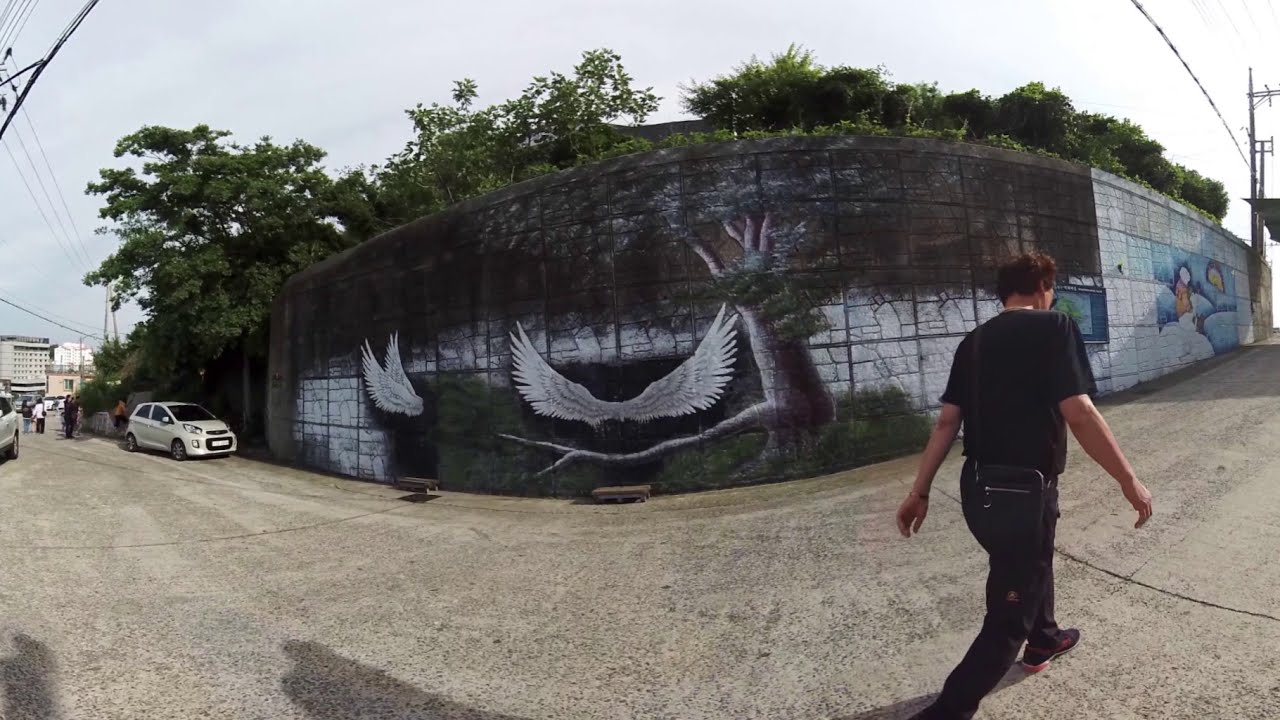This full-color photograph, taken outdoors on a sunny day, depicts a street scene with a horizontally rectangular composition. Dominating the image is a large stone or brick wall adorned with vibrant murals, including depictions of gigantic white birds in flight, likely representing angel wings, alongside painted trees. The wall is flanked by trees, one of which has a bare branch, adding a natural element to the urban setting. To the left, beyond the wall, stand gray buildings, partially visible, with a few people and white cars parked along the road.

In the foreground, a middle-aged man — characterized by his longer hair, aviator sunglasses, and a bracelet — walks away from the camera. He is dressed entirely in black, with a black t-shirt, black jeans, and black shoes with red soles, and he carries a satchel across his back. Further down the street, more murals can be seen, including one resembling a snow scene, as well as additional people and vehicles adding depth to the lively urban tableau.